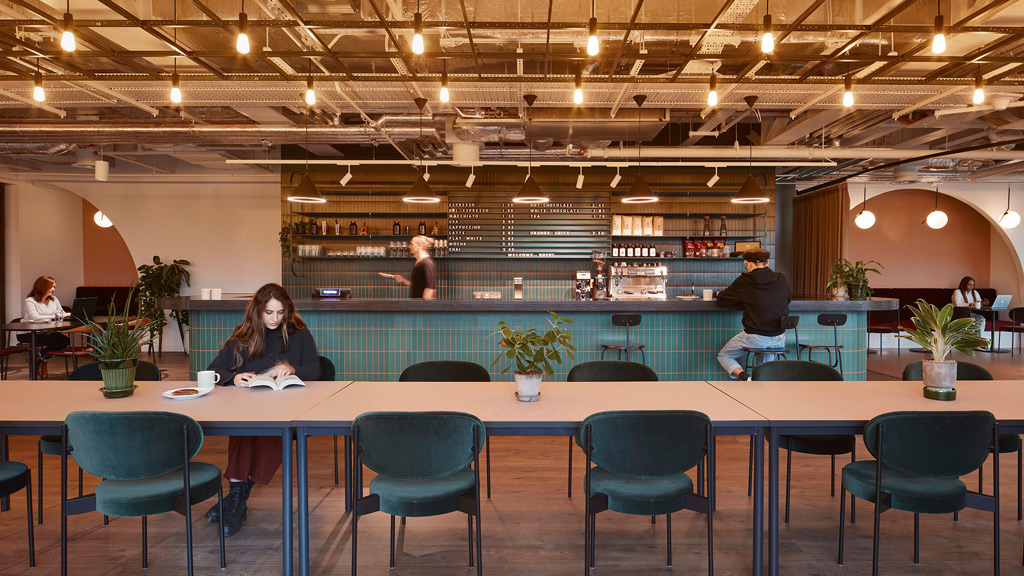The image is a color, horizontally-oriented photograph depicting a bustling cafeteria or dining hall, reminiscent of a university setting. The scene is anchored by a long row of beige-brown wooden tables with sleek, dark metal legs stretching across the bottom third of the image. Arranged along both sides of these tables are a mix of dark teal cushioned chairs and black cushioned chairs, some neatly tucked in while others are slightly slid out.  

In the foreground, a young white woman with long brown hair, dressed in a black sweater, sits on the left side of the table. She appears deeply engrossed in a book open in front of her on the table, her hands holding the pages down. Beside her book, she has a white cup of coffee and a saucer, adding a homely touch to the scene. Scattered strategically along the table are two or three potted plants, bringing a hint of nature indoors.

The background features a long, dark gray service counter that runs horizontally across the image. The counter is equipped with several black stool chairs, one of which is occupied by a man in a black shirt and jeans, seen from behind as he seems to be reading. Behind the counter, a white server in a black T-shirt is captured in profile, moving leftward within the frame. Overhead, industrial-style track lighting bathes the area in functional brightness.

To the right of the counter, there's an arched opening where another person is spotted, seated at a table, engrossed in their own activities. There’s a hint of a menu board in the background—black with white letters—though the text remains unreadable from this distance. On the far left, another alcove reveals yet another person focused on their studies, underscoring the dual purpose of the space as both a dining and study area.